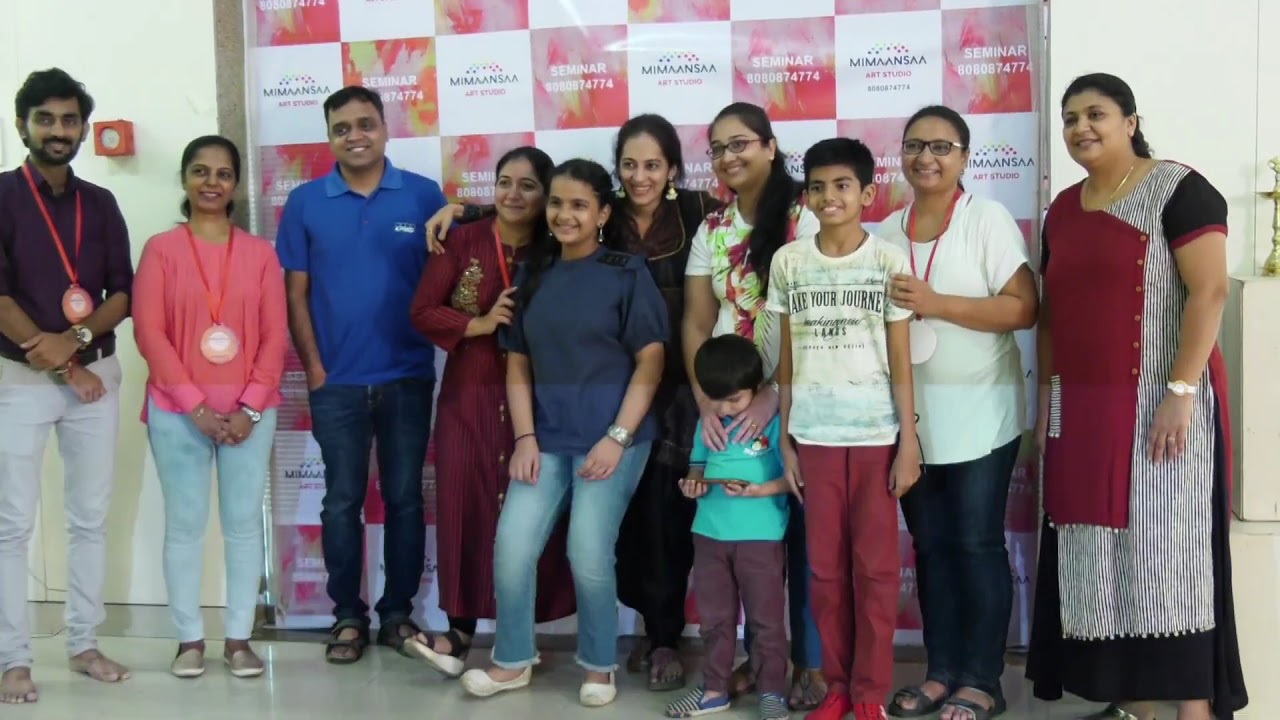The image depicts a group photo of eleven people consisting of eight adults in the back row and three children in the front. They are all smiling and facing the camera. Behind them is a checkered banner featuring a pattern of alternating white and pink (or red) squares. The pink squares display the words "seminar" along with some numbers, while the white squares read "Me Manasa" or possibly "Momenaso". The group is standing on a shiny, reflective floor, and they appear to be casually dressed, with one person on the far left notably barefoot. Most of the adults are wearing badges on lanyards around their necks, indicating that this photo was taken at a seminar or conference event. The participants’ attire ranges in color including pink, blue, purple, and white, adding a vibrant touch to the image.